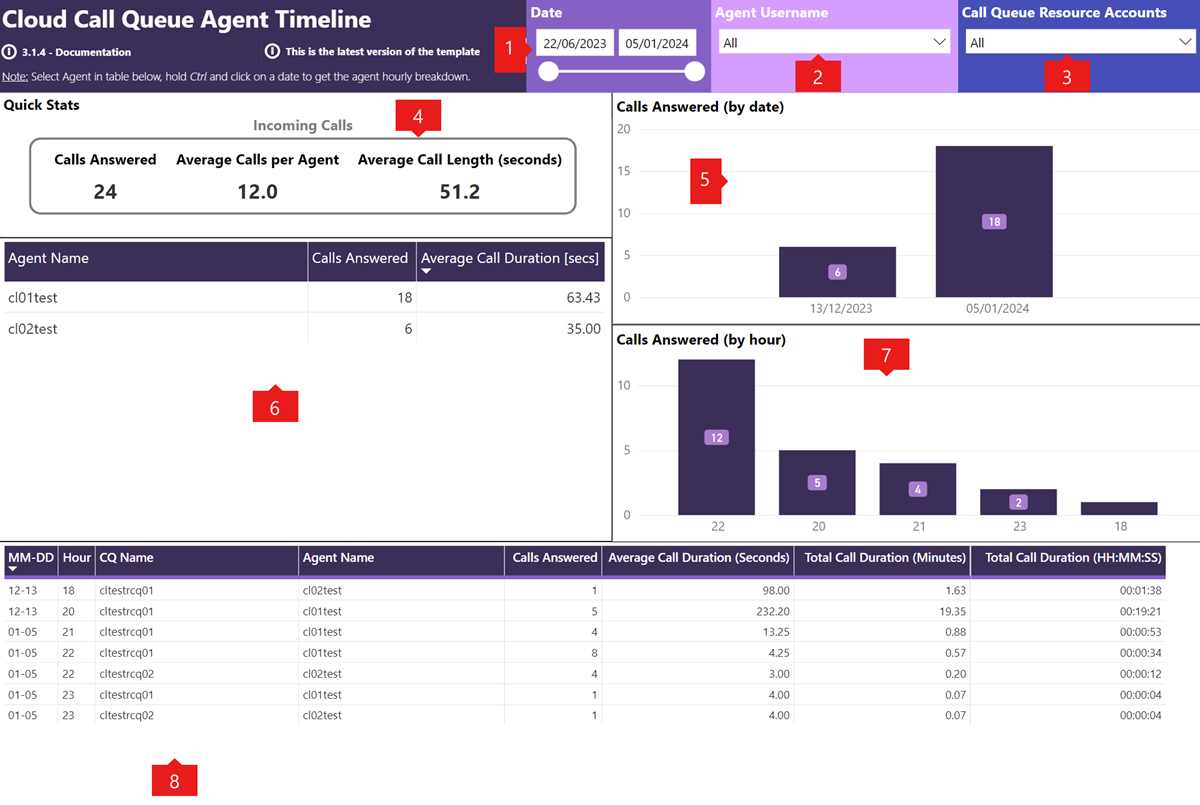The image is a detailed screenshot of a cloud-based call queue management software, specifically the **Cloud Call Queue Agent Timeline** version 3.1.4. At the top left, in a purple bar with lighter shades to the right transitioning to blue, the text confirms this is the latest version. The interface is highly data-dense, segmented into multiple areas, each annotated with red boxes numbered 1 through 8.

- **Section 1:** Displays the date range from June 22, 2023, to May 1, 2024.
- **Section 2:** Shows agent username with a dropdown menu, currently set to "All".
- **Section 3:** Indicates call queue resource accounts, again with "All" selected.
- **Section 4 (Quick Stats):** Presents quick statistics:
  - Calls answered: 24
  - Average calls per agent: 12
  - Average call length: 51.2 seconds
- **Section 5:** Contains a bar chart of calls answered by date, displaying data points such as December 13, 2023, and January 5, 2024.
- **Section 6:** Lists a table of individual agent names, total calls answered, and their average call durations.
- **Section 7:** Features another bar chart, this one showing calls answered by hour, with hourly variations such as 22, 21, and 18.
- **Section 8:** Provides a detailed log with a table format listing each call, including the date, hour, agent name, call time, and duration.

This comprehensive software seems tailored for call centers, offering detailed insights into agent performance, call traffic, and various analytics, with user instructions embedded for further breakdown of data.